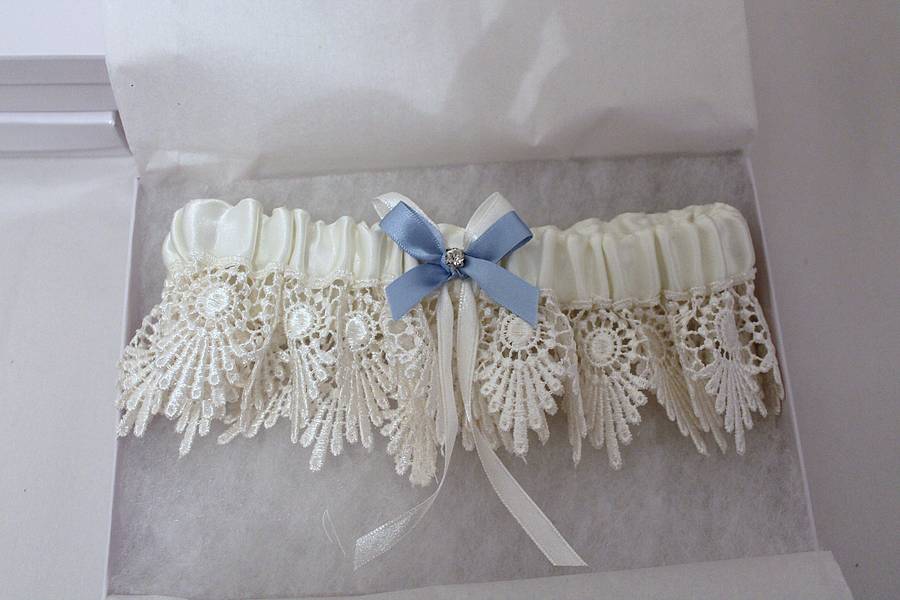This is a detailed color photograph of a ceremonial bridal garter, typically used in weddings. The garter is displayed inside a presentation box lined with soft white cotton-like material. The box is placed on a gray surface with a white backdrop. The garter itself features a gathered, rippled satin band that creates a textured appearance. At the top center of the band, a delicate white bow overlays a smaller blue bow, which is adorned with a tiny diamond-like stone. Two long white ribbons extend from this blue bow, gracefully curving outward, one to the left and one to the right. The bottom edge of the garter is trimmed with intricate lace, resembling floral patterns or lace doilies, adding to its ornate design. The entire arrangement is elegantly presented in the open box, creating a picturesque and detailed composition against the white and gray background.